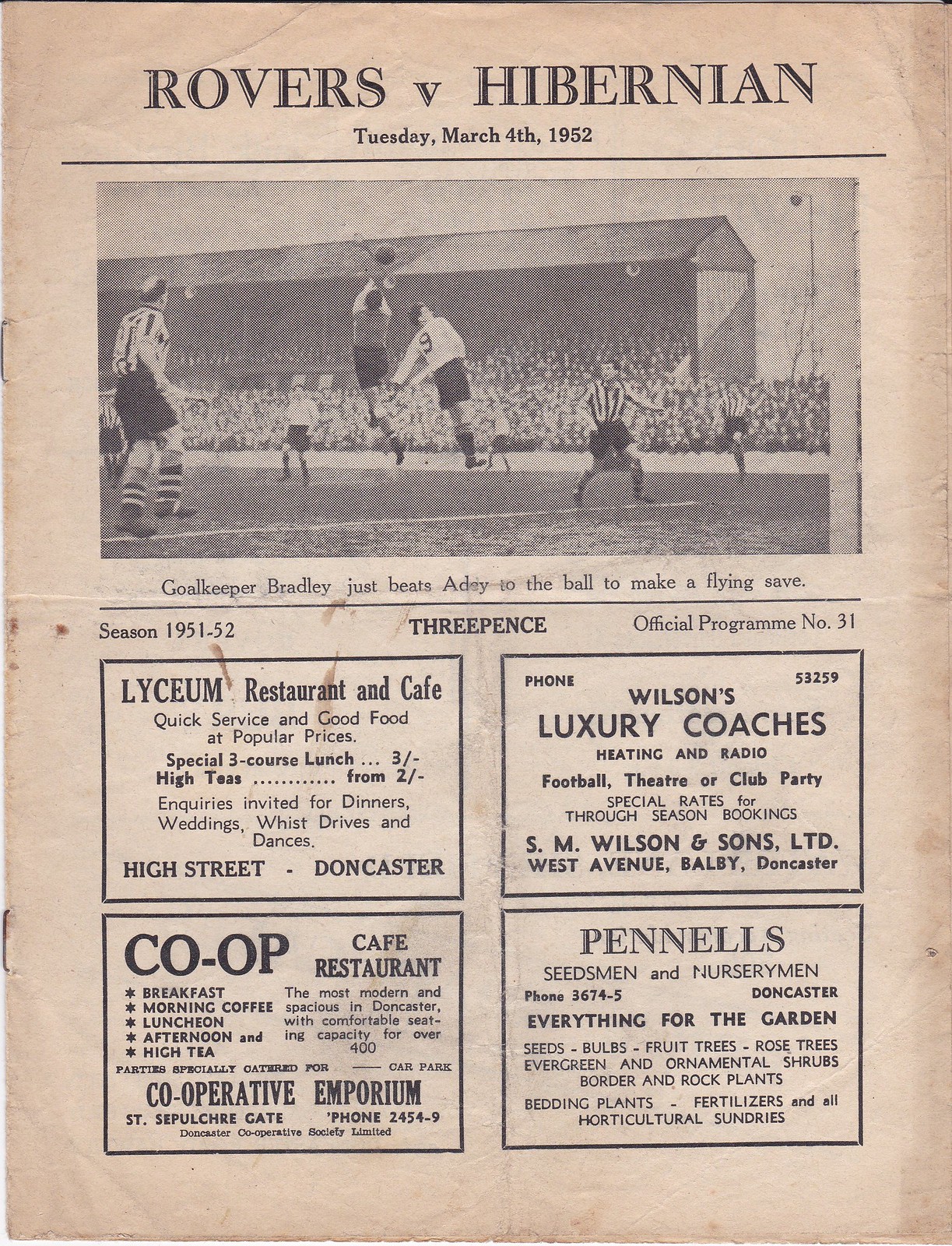This advertisement is for a historic soccer match between the Rovers and Hibernian, held on March 4th, 1952. The aged, tan-colored sports program is marked with dark spots, folds, wrinkles, and staples on the left side, indicating its vintage nature. The top of the program prominently features "Rovers versus Hibernian" in bold black letters, with the date clearly displayed beneath. Below the headline, a faded black-and-white photograph captures a dramatic moment on the field, where two soccer players are seen leaping into the air in a stadium setting. Additionally, the program includes four sponsorships: a luxury coach service, a Co-op Cafe Restaurant, a Lyceum, and a nursery, all printed in black lettering. The back of the program seems to recap a key play from the game, highlighting goalkeeper Bradley making a notable save by intercepting a ball, described as "goalcaptor Bradley bears Addy to a ball on him and makes a fine save."